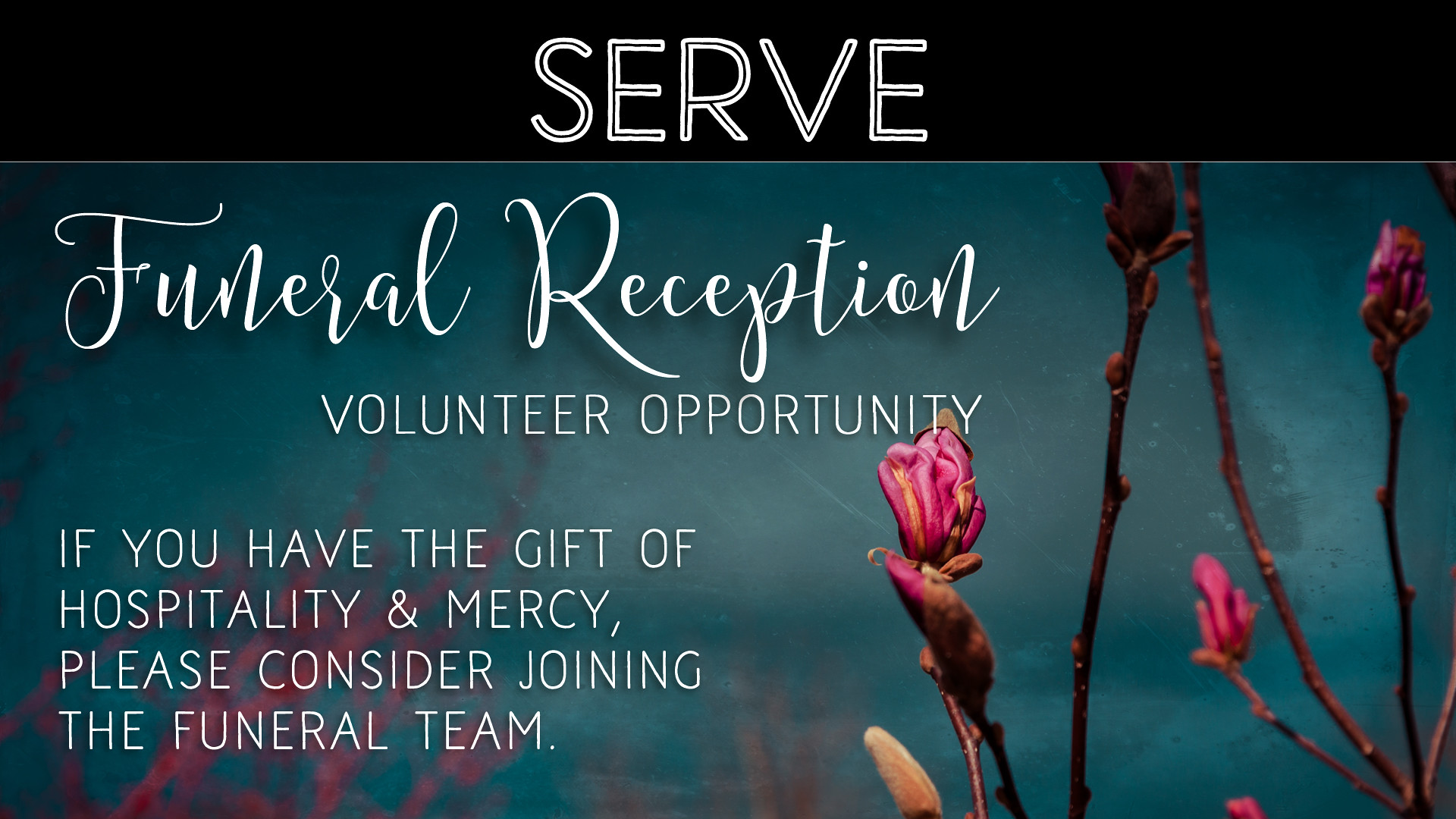The image features a prominent black top border with the word "SERVE" written in bold white letters, each letter intricately traced with fine black lines. Below this, the background transitions to a soothing blue, accentuated by delicate images of pink flowers. On the left side, sprigs and stems of the flowers extend upwards, while on the right, the blossoms are more fully visible. Directly beneath the word "SERVE," on the left side, the phrase "Funeral Reception" is elegantly written in large cursive white font. Just below that, more centrally aligned and in all capital letters, the text "VOLUNTEER OPPORTUNITY" appears in a straightforward print font. Skipping a few lines towards the bottom left corner, the text reads: "If you have the gift of hospitality and mercy, please consider joining the funeral team," spread across four lines, inviting viewers to participate.